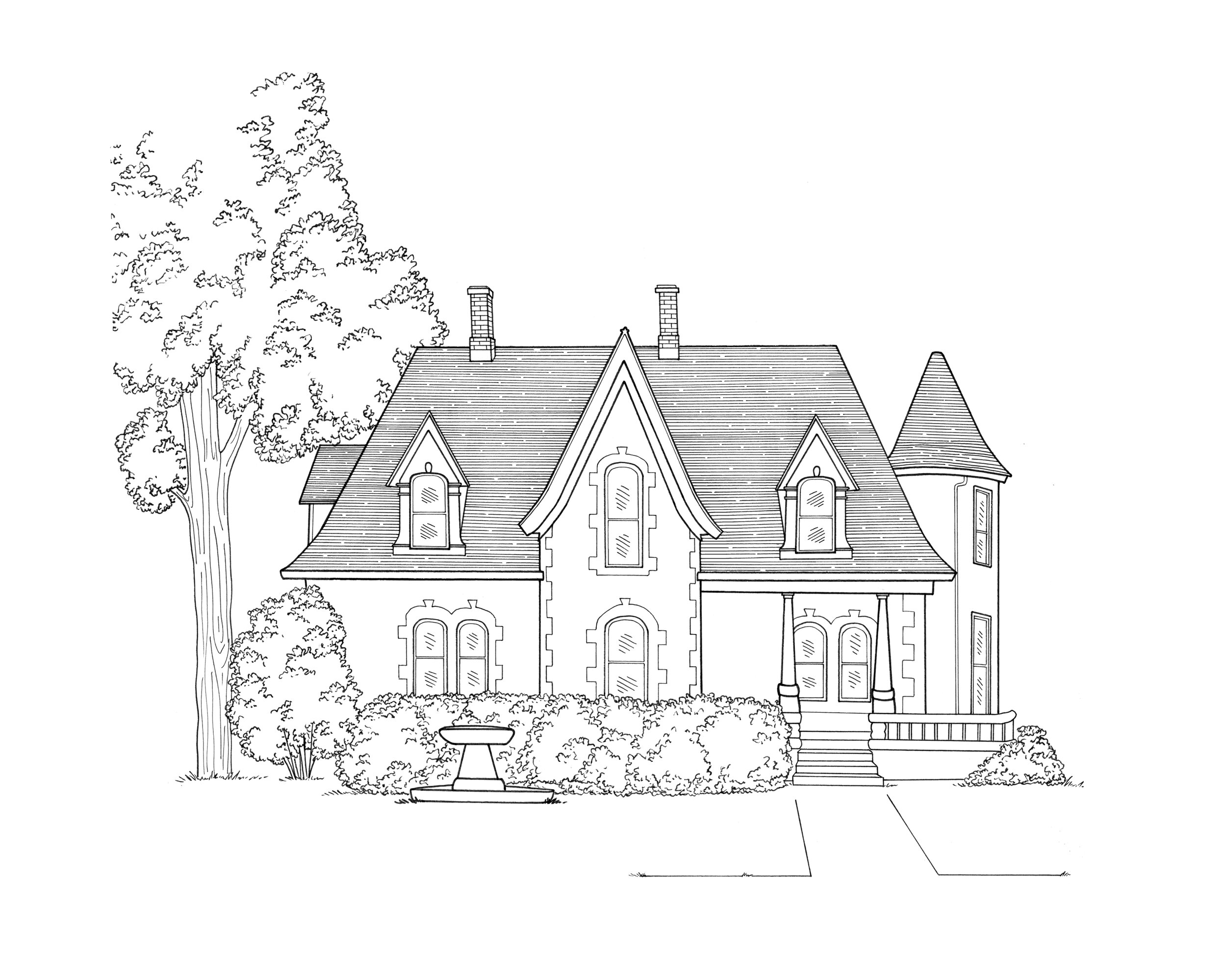This detailed pen-and-ink illustration or computer-assisted drawing of a two-story house showcases a blend of Tudor and Victorian architectural styles. The house features an intricately designed turret on the right, arched windows on both floors, and dormer windows on the roof, indicating a second floor comprised of three visible windows. The front facade includes a porch with two columns flanking the entrance and a small stairway leading up to it. Additionally, the design includes notable details such as two chimneys, a large tree to the left, smaller shrubs in the foreground, and a birdbath situated in front of the house. The overall composition, rendered in precise black lines on a white or transparent background, evokes a classic, old-fashioned aesthetic suitable for an architectural drawing or a coloring book.